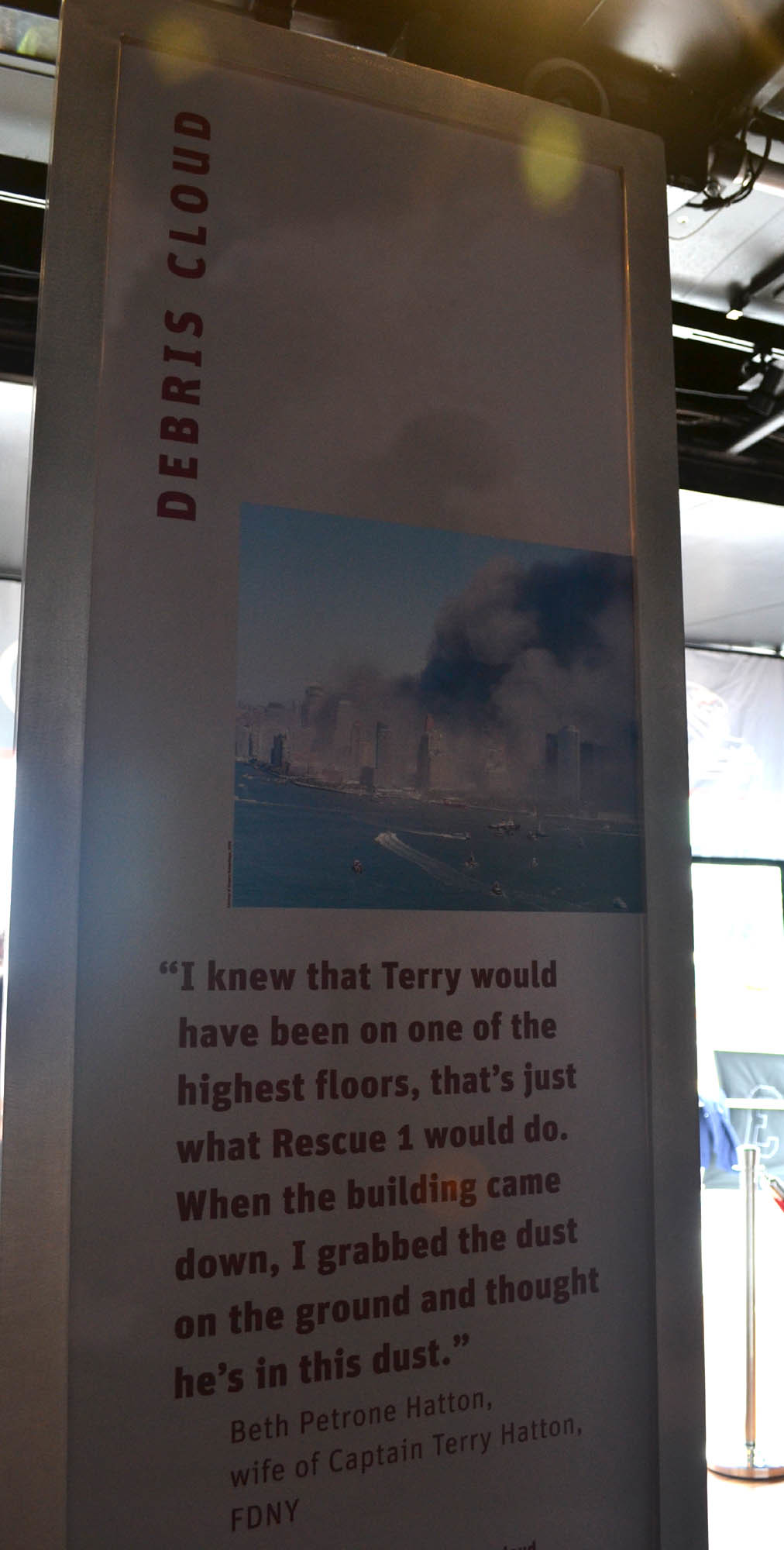This image captures a tall, vertical sign inside a museum, specifically as part of a memorial exhibit for 9/11. The sign prominently features the words "Debris Cloud" written vertically in red on the left side. In the center, a haunting photograph of the World Trade Center enveloped in a cloud of debris is displayed. Below the photograph, against a white background, is a poignant quote in red text from Beth Patron Hatton, wife of FDNY Captain Terry Hatton: "I knew that Terry would have been on one of the highest floors that's just what Rescue One would do. When the building came down, I grabbed the dust on the ground and thought, 'He is in this dust.'" The surroundings of the sign suggest it is part of an illuminated, expansive museum space dedicated to remembering the events of 9/11.